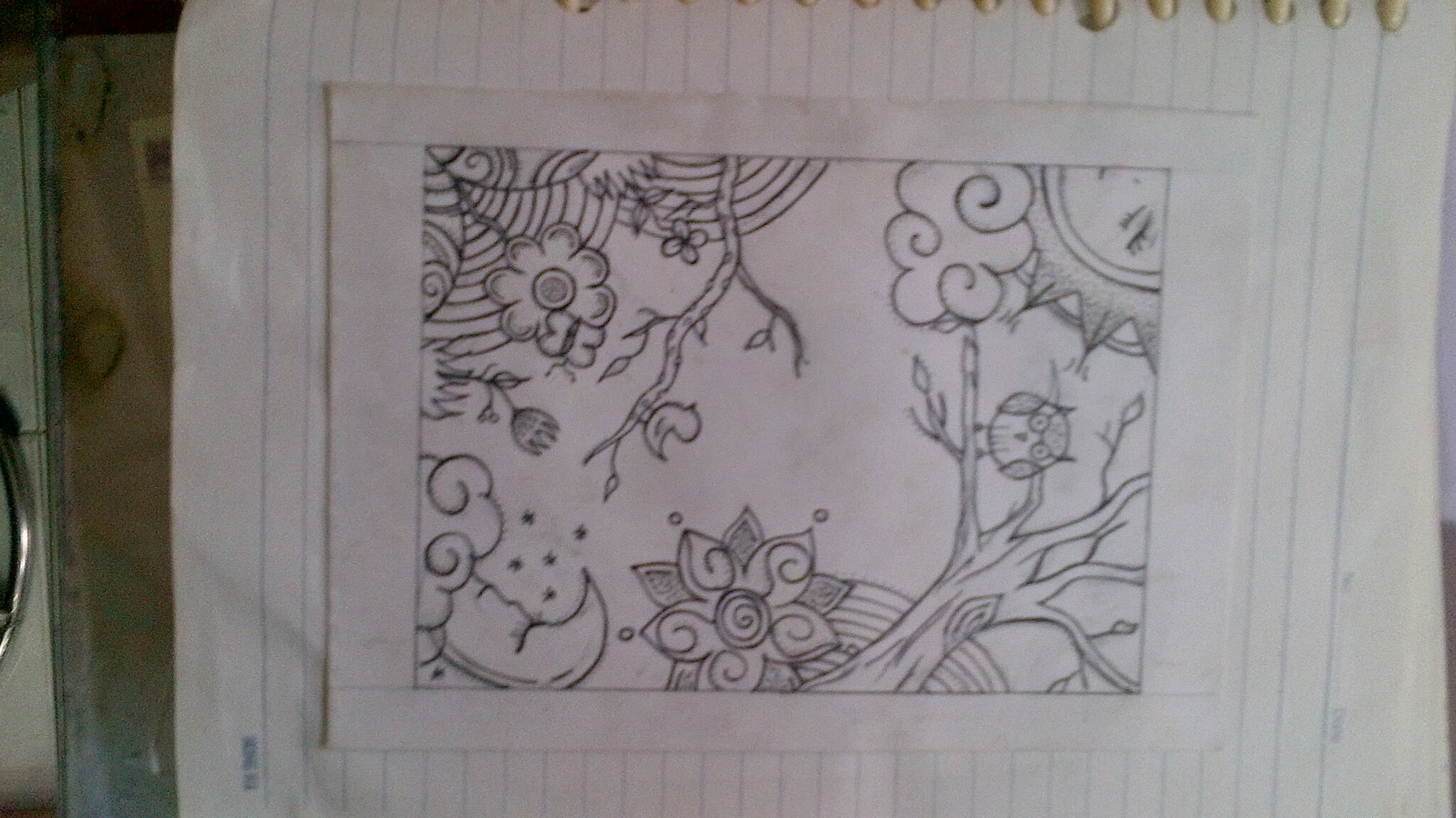The image is a photograph of a hand-drawn sketch on plain white paper, which is resting on an open spiral notebook with horizontally ruled pages. The notebook's spiral wires are visible at the top of the frame. The sketch is drawn in black ink and viewed from the side, making the orientations slightly off-kilter. The artwork itself is ornate and stylized, featuring various elements: a prominent tree trunk situated in the lower right-hand corner with a plump owl perched on it, looking straight ahead. In the upper left corner, there's a spider web with a flower growing out of it. The top of the drawing showcases part of a compass with surrounding clouds, while the lower left corner shows a crescent moon with eyelashes, giving it a sleepy appearance, enclosed by clouds and stars. Centrally at the bottom of the drawing, there is an ornate flower with intricate details. Additional features include a partial sun with eyelashes in the upper right, small branches, a little bird resting on a branch, and a butterfly hovering near another flower, all contributing to the rich and whimsical composition. The notebook and paper appear to be on a flat surface, possibly a tabletop.